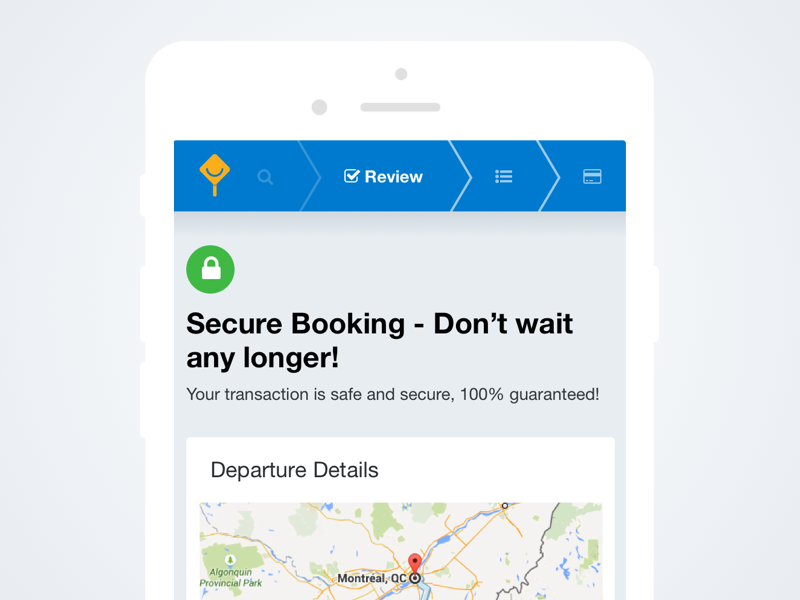This image captures the top portion of a phone screen, illustrated, not an actual phone screen, presented with a clearly defined white outline against a light gray background. Occupying the uppermost section is a vibrant blue bar, prominently featuring a yellow diamond-shaped icon on the far left. Adjacent to this icon is a magnifying glass representing the search function. The white text near the search icon reads "Review," prefaced by a checkmark symbol, indicating a confirmation or completion status. 

On the right side of this blue bar, aligning towards the edge, is a hamburger menu icon signifying additional options, and a credit card icon suggesting a financial transaction or payment method. 

Beneath this blue bar filled with icons lies a primary screen area displaying impactful, reassuring text: "Secure booking, don't wait any longer. Your transaction is safe and secure, 100% guaranteed." Below this assurance-based message, the image shows the upper half of a map focused on the Algonquin Provincial Park area, marked with a pin indicating a location in Montreal, Quebec. Above the map, the text "Departure details" serves as a heading, likely categorizing the map content or emphasis on relevant travel logistics.